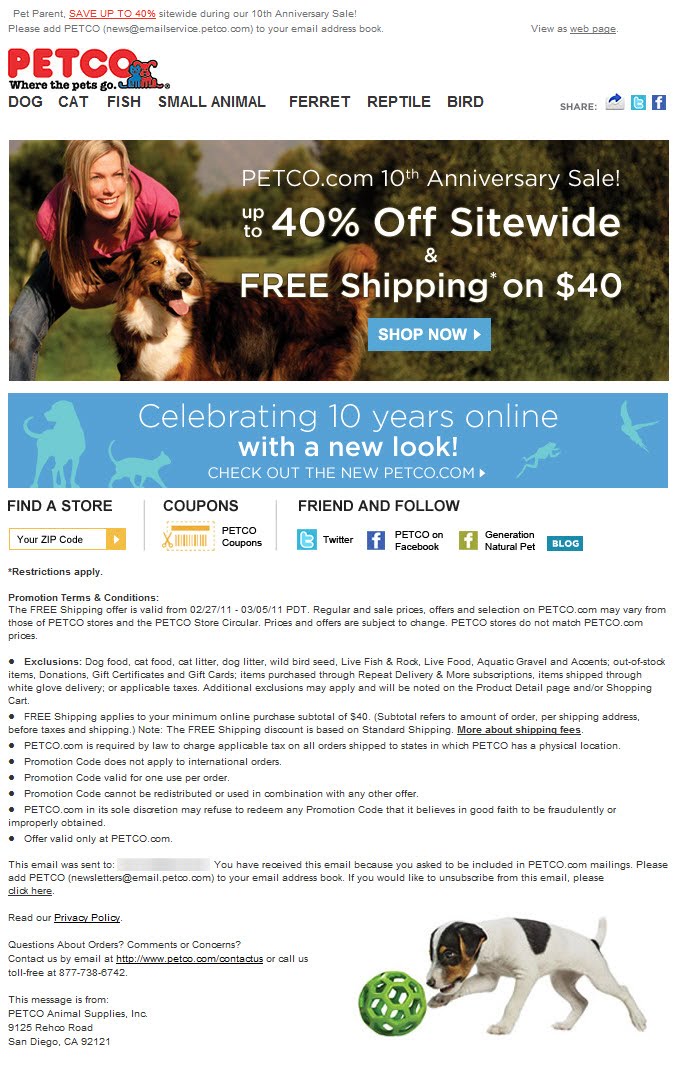The main page of Petco’s website is vividly designed to engage pet lovers. At the top left-hand side, the familiar Petco insignia features a blue cat and a red dog. Below the logo, black text menus direct users to various pet categories: Dog, Cat, Fish, Small Animal, Ferret, Reptile, and Bird.

An eye-catching advertisement showcases a smiling woman with blonde hair wearing a pink shirt, playing outside with a Border Collie. The ad, celebrating Petco.com’s 10th anniversary sale, boasts up to 40% off site-wide and free shipping on orders over $40. A prominent blue “Shop Now” button invites users to take advantage of these offers. The slogan “Celebrating 10 years online with a new look. Check out the new Petco.com” emphasizes the website's modernization.

On the right-hand side, users can find a store locator featuring a yellow zip code finder, and options for Petco coupons. The page highlights Petco’s social media presence, including links to their Twitter and Facebook pages, the “Generation of Traditional Pet” blog, and connections to friends and followers.

In the bottom right-hand corner, a playful puppy is pictured enjoying a hollowed-out green ball. The footer of the page contains textual information about restrictions, terms and services, and promotional code applicability, noting that international orders are excluded from the promotion. 

Overall, the webpage combines lively visuals and detailed information, creating an inviting and informative experience for pet enthusiasts.